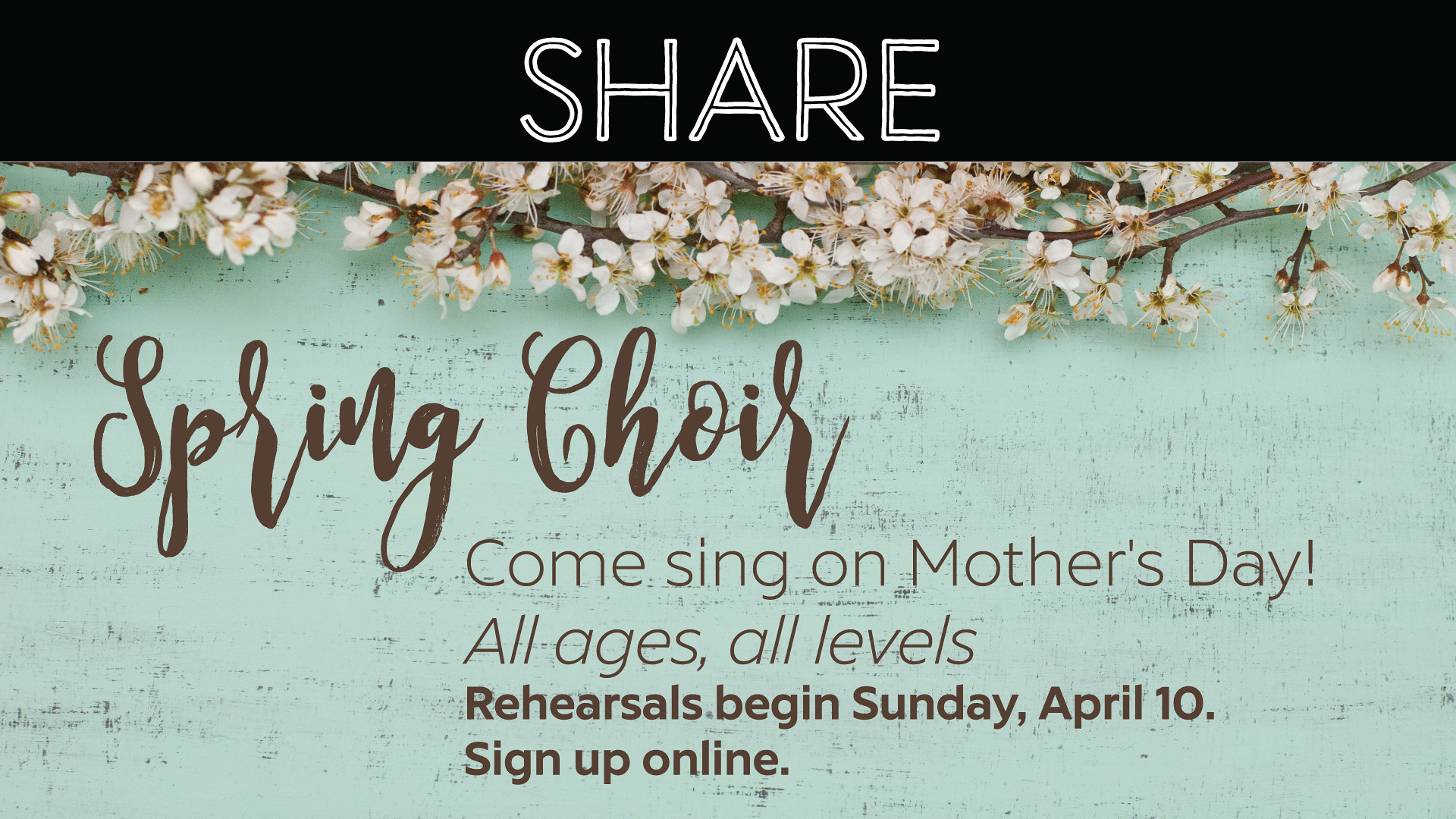The image appears to be an event notice designed for digital sharing, resembling a business card. It is a rectangular scan, about twice as wide as it is high, with no borders or links. The design is divided into two sections. The top section is a black banner occupying less than one-fifth of the image's height, featuring the word "SHARE" in white capital letters. Below the banner, the main section displays a worn green, slightly weathered wall with darker shades showing through. At the top of this wall, white flowers on branches are depicted, adding a touch of elegance. In the center of this section, "Spring Choir" is written in cursive purple font. Beneath this, in plain font, the text reads: "Come Sing on Mother's Day! All ages, all levels. Rehearsals begin Sunday, April 10th. Sign up online."